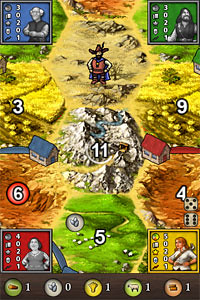This screenshot captures an outdoor scene from an older video game, characterized by its vivid colors and pixelated graphics. Dominating the center of the screen is a figure clad in a red top, sporting a cowboy hat and a cape, confidently standing with hands on hips. Surrounding this figure are various playful elements, including a small cartoon house with a blue gabled roof and another similar house with a red roof. The image features a mixture of yellow, orange, and green hues, with a prominent white area in the center drawing the viewer's attention. In each of the four corners, there are avatars representing different characters, both male and female, each displayed within a colored box accompanied by numerical values, hinting at their stats or levels. The nostalgic artwork and design elements emphasize the game’s retro origins.